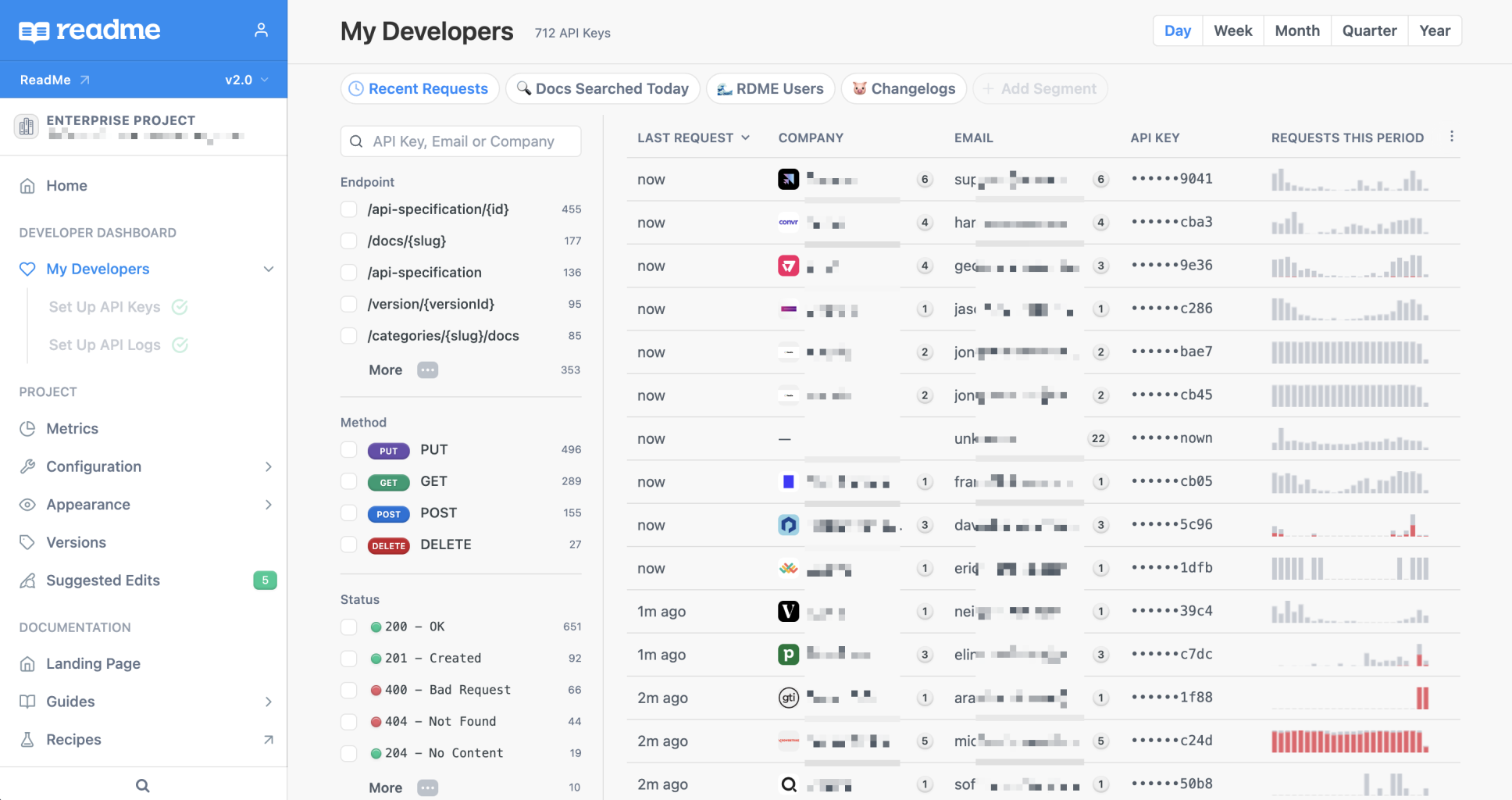The image depicts a detailed view of the "Read Me" website, specifically focusing on its interface and available features. 

In the upper left corner, there is a blue box containing the website’s name, "Read Me," accompanied by a small person icon that likely serves as an account access point. Directly below this, the text "Enterprise Project" appears, though it is blurred out. Following this, the menu lists "Home" as the main category, under which the "Developer Dashboard" is found. The "Developer Dashboard" menu features three highlighted subcategories: "My Developers," "Setup API Keys," and "Setup API Logs." The "My Developers" subcategory is currently highlighted in blue and marked with a heart icon.

Next in line is the "Project" category, encompassing subcategories such as "Metrics," "Configuration," "Appearance," "Versions," and "Suggested Edits." Subsequently, the "Documentation" category lists subcategories like "Landing Page," "Guides," and "Recipes." Below this, a magnifying glass icon signifies a search function.

The main content area prominently displays "My Developers" with a total of "712 API Keys" listed. In the upper right corner of this section, options for different time frames—Day, Week, Month, Quarter, and Year—are available, with "Day" currently selected and highlighted in blue.

Below this, a section titled "Recent Requests," also highlighted in blue, presents various data categories such as "Docs Search Today," "RDMI Users," and "Channel Logs." Another segment follows, showing "Endpoint" with related subcategories that appear to be files. The adjacent "Method" section categorizes entries by HTTP methods: "Put" (purple), "Get" (green), "Post" (blue), and "Delete" (red). Following this is the "Status" category featuring various clickable elements which seem to be numbers, possibly files.

The main image further details the different files, showing when they were last requested, the company names (though blurred), emails (also blurred), and API keys. Additionally, there is a section specifying "Requests This Period."